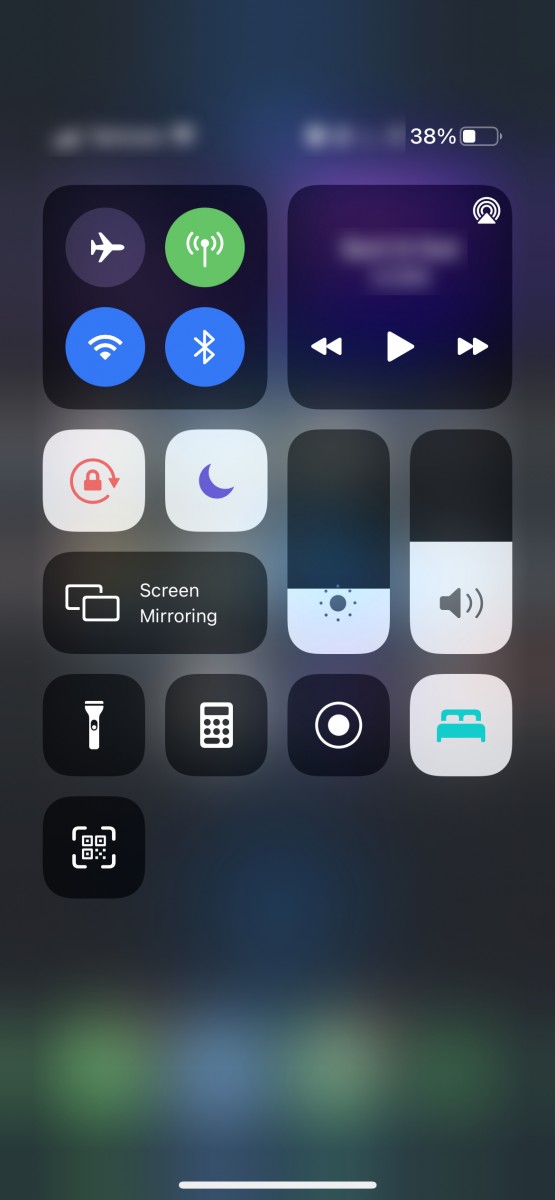This screenshot captures the Control Center of an iPhone, showcasing a variety of essential settings and controls. The battery level is clearly visible at 38%, indicating that the device is not currently charging. 

In the top-left section, there is a square grid of four primary buttons: Airplane Mode, Cellular Data, Wi-Fi, and Bluetooth. Each icon is neatly arranged for easy accessibility. 

In the upper-right section, music playback options and volume control sliders are displayed, offering control over media and sound levels. The volume is set to approximately 50%.

The middle section reveals additional settings: Orientation Lock is activated, and Do Not Disturb mode is enabled. A Screen Mirroring option is present but currently inactive. 

On the right side, there are sliders for adjusting brightness and volume. The brightness is set to about 30%, while the volume stands at around 50%. 

The bottom section contains a row of functional icons: Flashlight, Calculator, Screen Recording, and Bedtime Mode. In the bottom-left corner, a QR code scanner icon is prominently placed for quick access. 

Overall, this snapshot of the iOS Control Center exemplifies a well-organized interface that provides quick access to frequently used settings and controls.